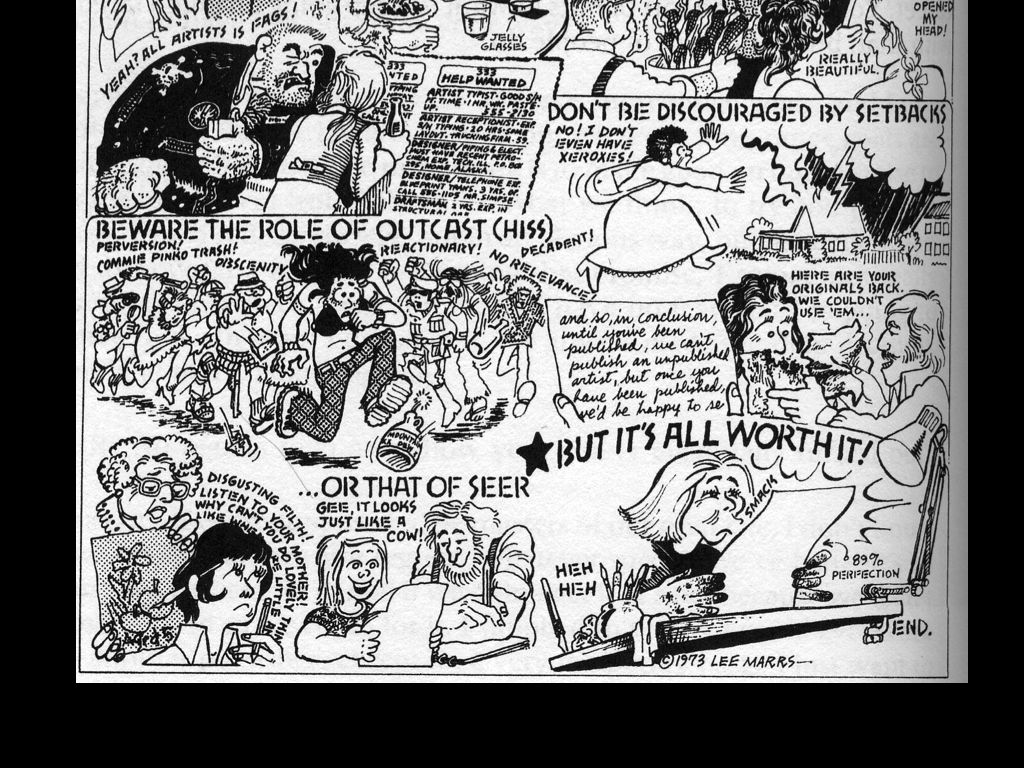This detailed comic art, titled with a copyright from 1973 by Lee Marrs, comprises a sheet of numerous busy and intricate panels set in a black and white style reminiscent of late 60s and early 70s Stoner Era art. The work narrates the struggles and resilience of an artist's journey through a series of vignettes. A recurring theme is perseverance despite adversity. In one panel, a character runs toward a burning house, lamenting the lack of Xeroxes for their work, symbolizing lost art. Another panel features a mob casting a hippie freak, yelling words like "reactionary" and "commie." Yet another panel shows an intimidating soldier proclaiming disdain for artists. One lower panel presents a teacher declaring an artist's work as "disgusting filth" and questioning why the student can't produce lovely things. The bottom tier, more legible, captures a pivotal moment: an artist with ink-stained fingers, indistinguishably gendered, affectionately kissing a piece of paper with a star and the words "it's all worth it" and an arrow indicating "89% perfection." This visual narrative encapsulates the trials, setbacks, and eventual triumphs of the artistic journey, underscored by the artist's signature in the lower right-hand corner, affirming the creation from over 50 years ago.